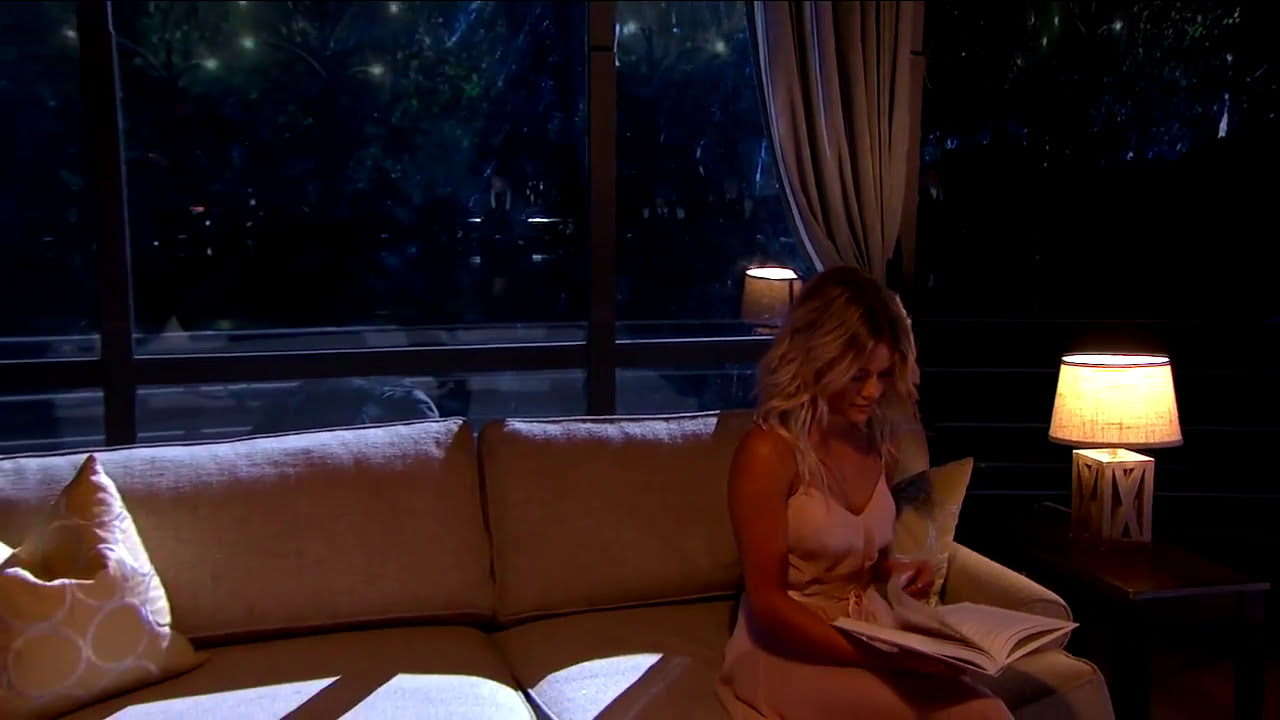In the nighttime scene set inside a living room, a beautiful blonde woman with hair cascading slightly below her elbows sits gracefully on a light peach-colored couch. She is deeply engrossed in a book placed on her lap, and she is dressed in a white or perhaps light pink dress. To her left stands a wooden side table topped with a lamp that has a round, white shade and an X-shaped design on its base, casting a warm glow perfect for reading.

Behind her is a large window with metal bars dividing it into multiple glass panels, partially veiled by a pulled-back brown curtain. Through the window, the dark night is visible, marked by scattered white spots that resemble stars or reflections, and shadowy leaves on branches. Adding a cozy touch to the setting, there are a couple of pillows on the couch; one is brownish, while another has a circular design pattern. The room's ambiance is ethereal, almost cinematic, highlighted by the faint glow that seems like moonlight or a photographer's flash, adding to the scene's serene and picturesque quality.